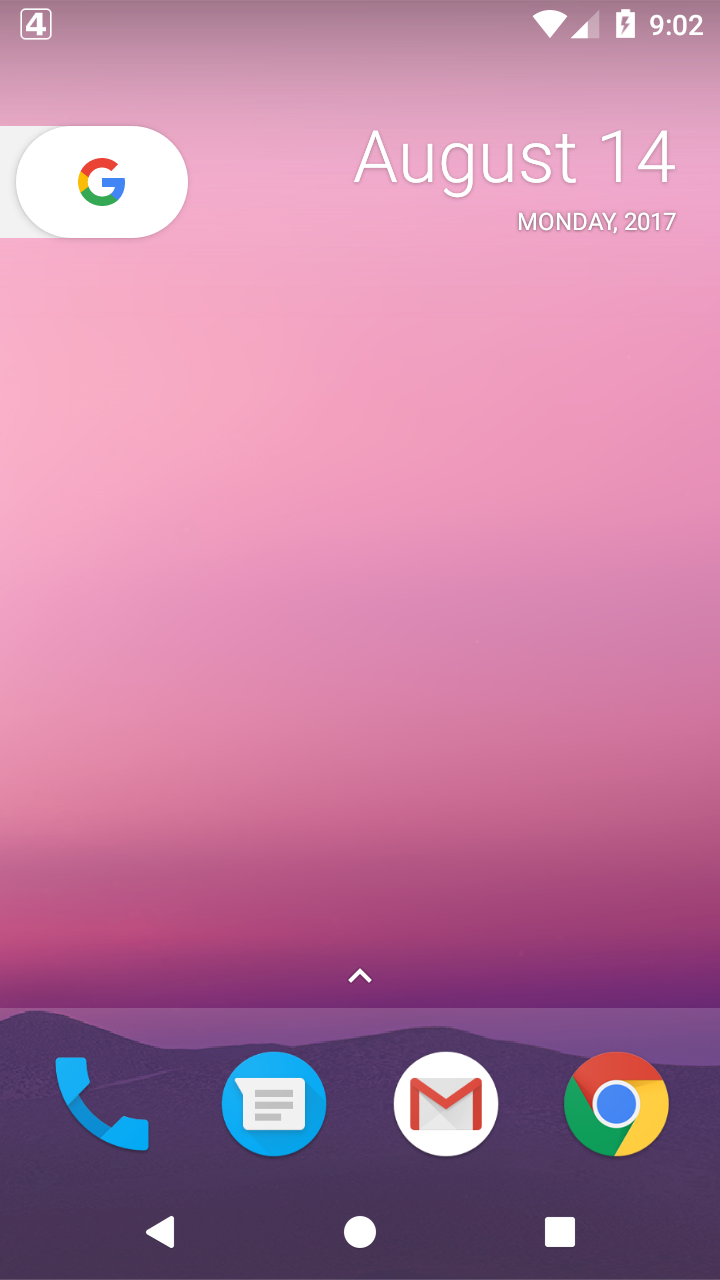The screenshot captures the home screen of a smartphone, showcasing various features and elements. In the top left corner, a large '4' is visible, though its significance is unclear. The top right corner displays the device's connectivity status, indicating two out of four Wi-Fi bars and a fully charged battery currently being charged (denoted by a lightning symbol). The time reads 9:02, with no indication of AM or PM.

The background showcases a gradient from pink at the top to purple at the bottom. Below the time display, which states "August 14th, Monday 2017," there is a Google search bar widget, suggesting a slide action for additional functionality. At the bottom of the screen is an upward-pointing arrow, hinting at expandable options or additional icons.

The bottom row contains four icons representing commonly used applications: a phone icon for calls, a messaging app, Gmail, and Google Chrome. Additionally, navigation buttons are visible, including a back arrow, home button, and an overview button for accessing all open tabs.